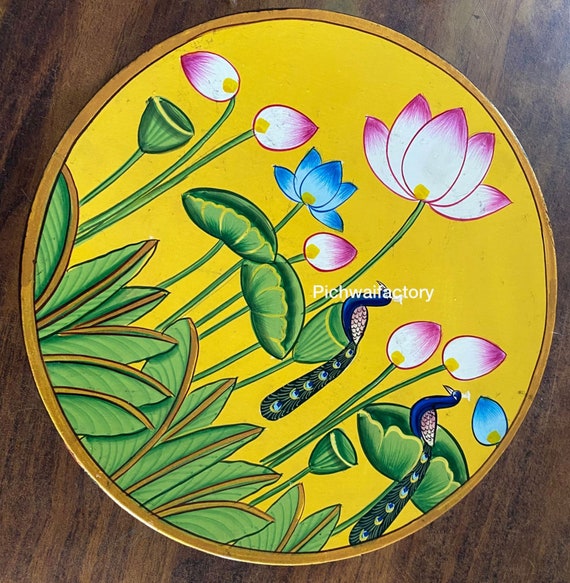This photograph captures a round, ornately decorated plate placed on a medium brown, wood-grain table. The plate features a vivid, golden-yellow background with a thin, golden border. At the bottom, green leaves spread out, providing a perch for two dark blue peacocks with distinctive peacock tails adorned with famous blue eye-spots. The birds are facing different directions, adding a dynamic touch to the scene.

Above the leaves, vibrant flowers with yellow centers and petals in shades of pink, white, blue, and purple cascade upward. The central area includes prominent purple, bell-shaped flowers accented by smaller blue flowers. Surrounding these main elements, the intricate artwork blends bright and lively colors, showcasing the hand-drawn quality of the design. Overall, the image presents a beautiful fusion of nature and art, perfectly framed by the natural finish of the wooden tabletop.